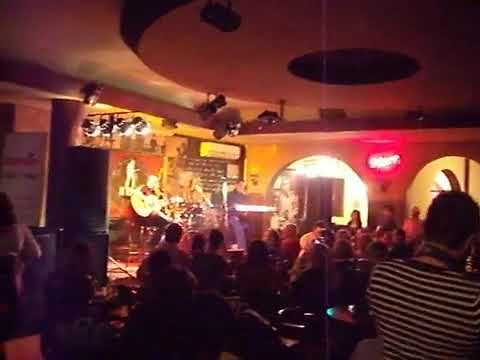In a dimly lit restaurant with yellow and white walls, the focus is on a small stage illuminated by overhead stage lights from the left side of the image. A musician, dressed in black pants and a red shirt, is seated on a stool, strumming a light brown acoustic guitar. The stage, which suggests an intimate setting akin to an open mic night, has a microphone positioned before the performer. To the right, multiple patrons are seated at round tables adorned with glass bottles and plates of food, attentively watching the performance. A person wearing a black and white striped shirt with a black strap around their neck is visible in the bottom right corner. At the center of the image stands a pillar, sporting a red neon sign, casting a soft red glow that subtly blends with the ambient light and shadows, contributing to the cozy yet vibrant atmosphere of the venue.